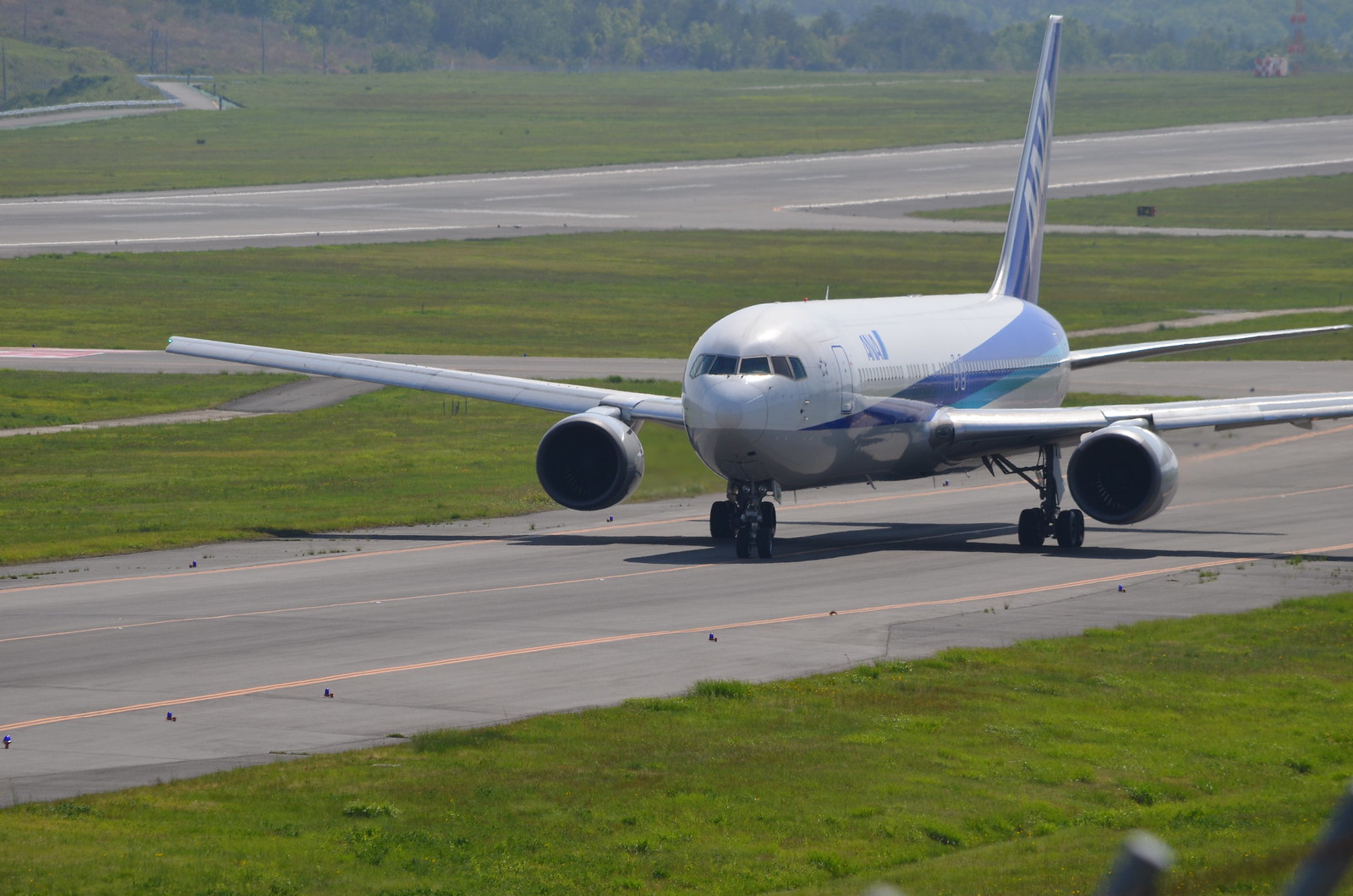This detailed photograph captures a white and blue ANA Airlines passenger jet centered on an airport runway. The aircraft, which appears to be a single-deck plane with the distinctive "ANA" logo, is positioned nose-forward, moving toward the viewer from the right perspective. Its body features a white top with a turquoise and dark blue diagonal stripe, complemented by dark blue stripes with white detailing on the tail. The plane sits firmly on the tarmac, where red-painted yellow lines guide its path, flanked by green grass. In the background, short grass fields stretch towards a border of trees, and connecting taxiways intersect the primary runway, contributing to the scene's bustling airport atmosphere.